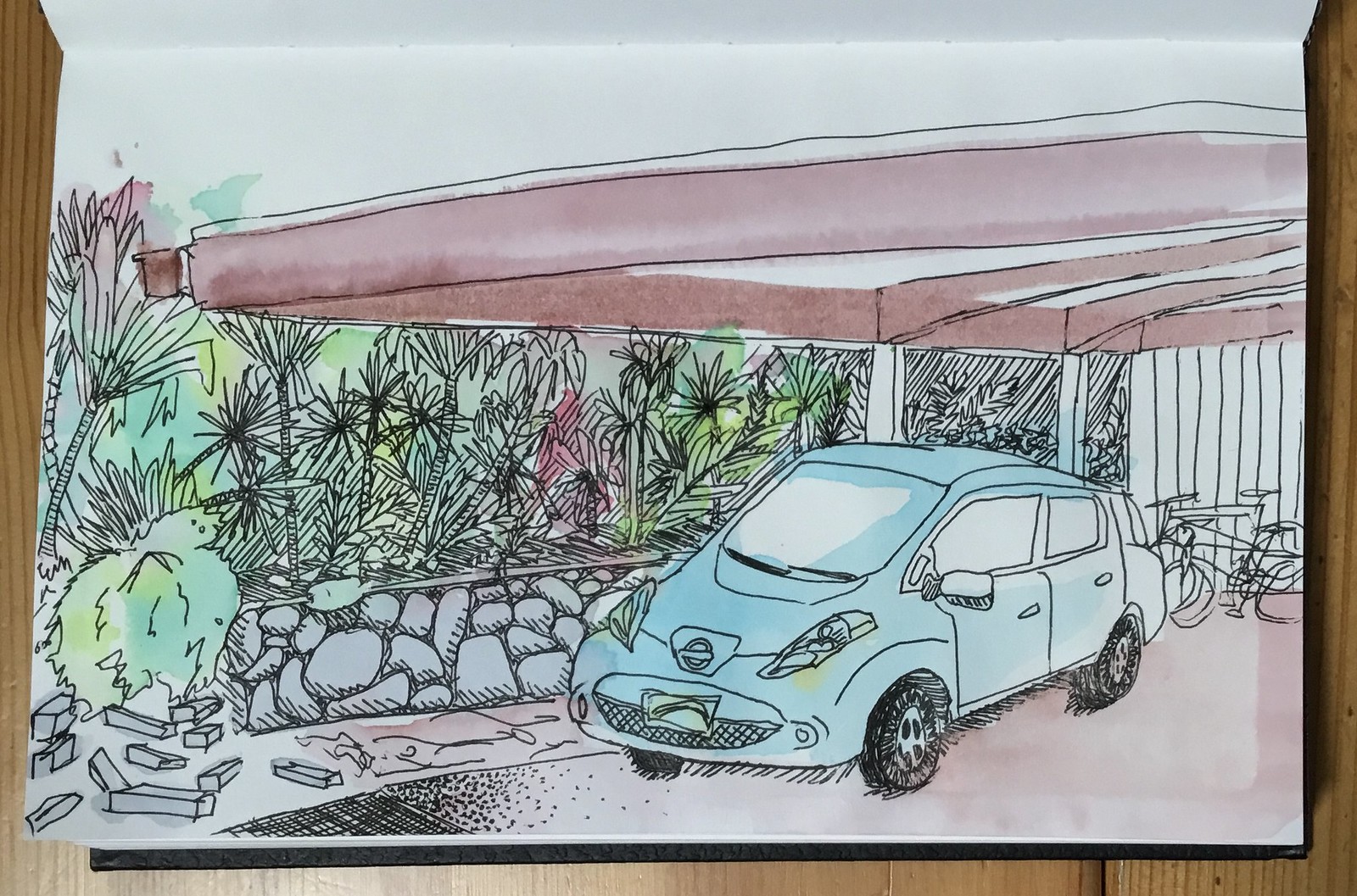A detailed pen and ink sketch, enhanced with delicate watercolor, captures the serene charm of a California-style carport. Resting against a wood grain surface, the illustration appears as a page in an artist’s sketchbook, framed by the book’s binding. The carport itself shelters a subcompact car, adorned with a prominent Nissan logo and modern headlights. The scene includes a small paver area and a miniature boulder retaining wall, with scattered bricks suggesting ongoing work.

Lush tropical plants, including small ferns and palm trees, add a touch of greenery to the tableau. Further back, bicycles lean against vertical lines, adding depth and interest. The carport's roof, complete with detailed struts, cross pieces, and even rain gutters, showcases the artist’s meticulous attention to construction elements. The watercolor wash brings the entire scene to life with soft pastels and serene seafoam blues, creating a harmonious balance between the detailed pen work and the gentle color palette. This small but captivating piece turns a simple moment into a tranquil masterpiece.